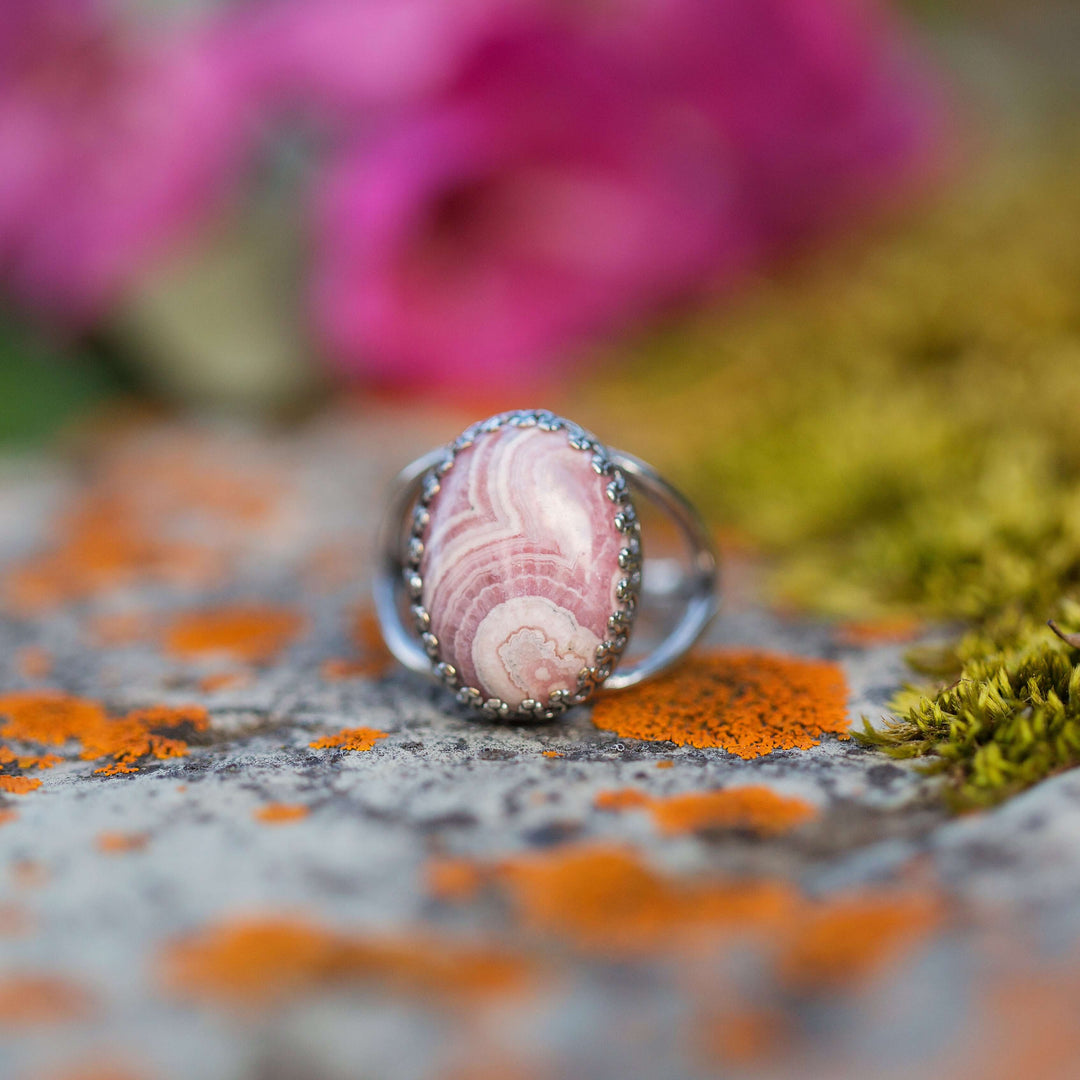This detailed photograph captures a close-up shot of a silver-colored ring laying on a cement or gravel pathway outside. The ring is adorned with a large, oval pink and white stone, featuring a delicate scalloped edge that forms a sort of halo around it. The camera focuses intently on the ring, leaving the background in a soft, artistic blur. Surrounding the ring on the ground are noticeable orange specks and patches of moss. The out-of-focus background hints at various colors, including greens that suggest grass and bright pinks and purples, likely indicating flowers. This expertly blurred backdrop contrasts beautifully with the sharply detailed ring, making it the clear focal point of what could be a striking advertisement for this stunning piece of jewelry.